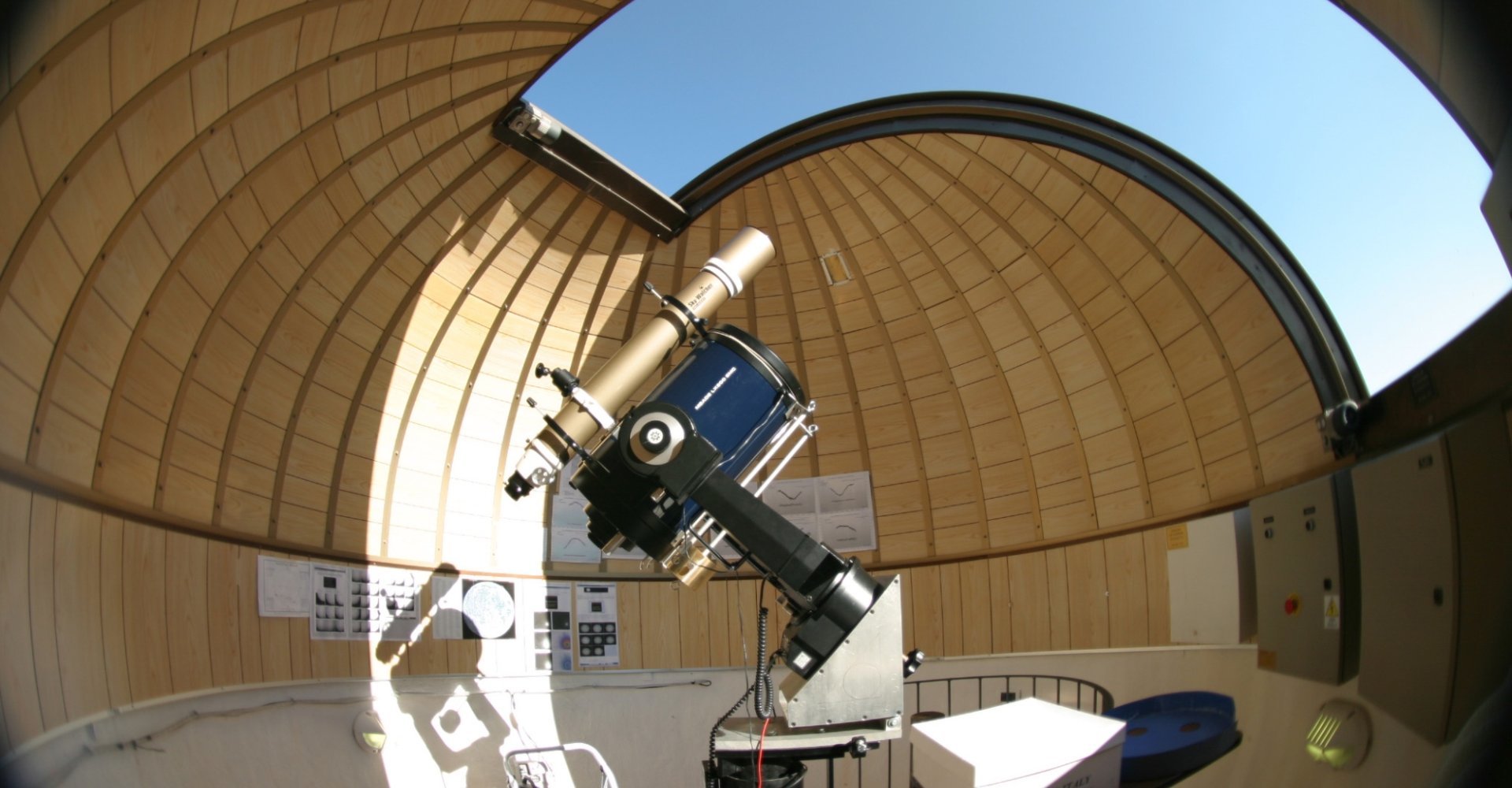The image captures the interior of a dome-shaped observatory, characterized by its light brown walls and an open ceiling that reveals the sky above. The focal point is a sophisticated telescope setup positioned centrally, featuring two distinct cylindrical components. The smaller, upper telescope, crafted from metal, is angled and adorned in a golden hue. This telescope is mounted on a substantial, dark stand that also supports a larger, stouter cylinder in dark black and blue tones. The stand and telescopes form an impressive array, angled upwards toward the opened ceiling. Numerous lens adjustments are visible on the apparatus. To the left, the background displays several pictures affixed to the wall, while soft sunlight casts intricate shadows across the scene, enhancing the observatory's tranquil ambiance.